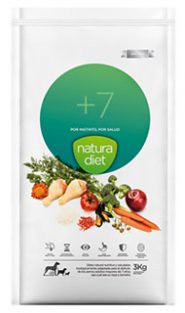A detailed, clean caption for the described image:

A color photograph of a white bag of dog food set against a pure white background. The focal point of the packaging is a large green circle situated in the upper middle portion of the bag with the text "+7" prominently displayed within it. Inside this green circle is a smaller, subsidiary circle that bears the brand name "Natura Diet" in white lettering. Below this central design, a vibrant, angled image of various nutritious foods stretches across the bag. The imagery includes chicken, carrots, a tomato, an apple, and some green leafy vegetables, with the left side of the image positioned slightly higher than the right. At the bottom left corner of the bag, there are artistic, monochromatic drawings of three dogs in different sizes. Additionally, there is text in dark ink towards the lower portion of the bag, but the specific wording is not legible in this view.